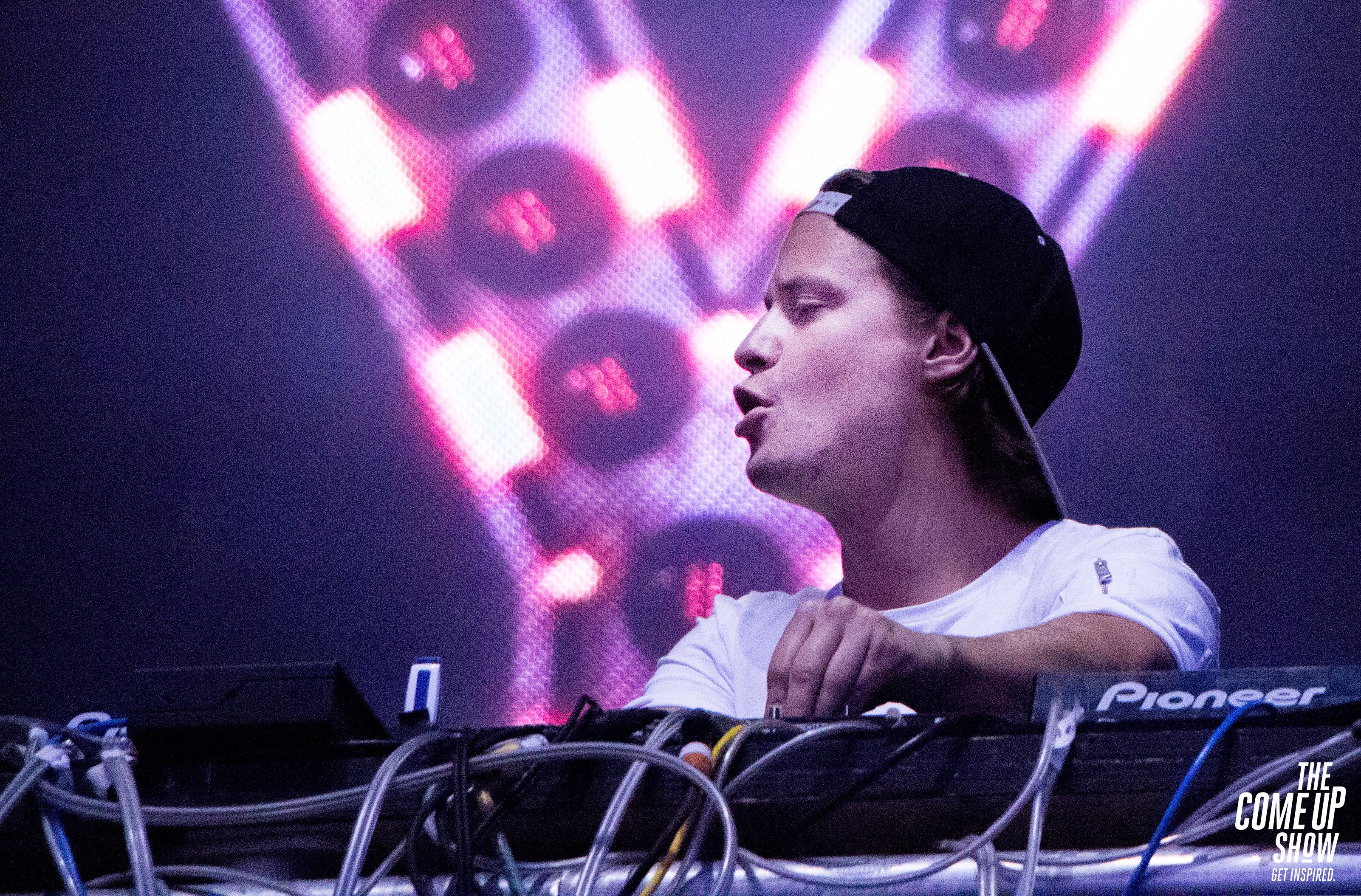The image features a white male DJ positioned behind an array of black Pioneer stereo equipment, distinguished by a prominent white "Pioneer" logo. The DJ is dressed in a white short-sleeve t-shirt and a backwards black cap with a grey or light blue brim, revealing the plastic snapback part. He is captured in the middle of a performance, with his left hand adjusting knobs and his mouth open, possibly speaking or making an expressive gesture. Only his upper body is visible, along with a tangle of white, blue, and yellow cords connecting to the mixer. The background is primarily dark but features a striking array of lights forming a Y-shape, with black circles and red lights at the center, adding a dynamic ambiance to the scene. In the bottom right corner, the text "The Come Up Show Get Inspired" appears overlayed in white.